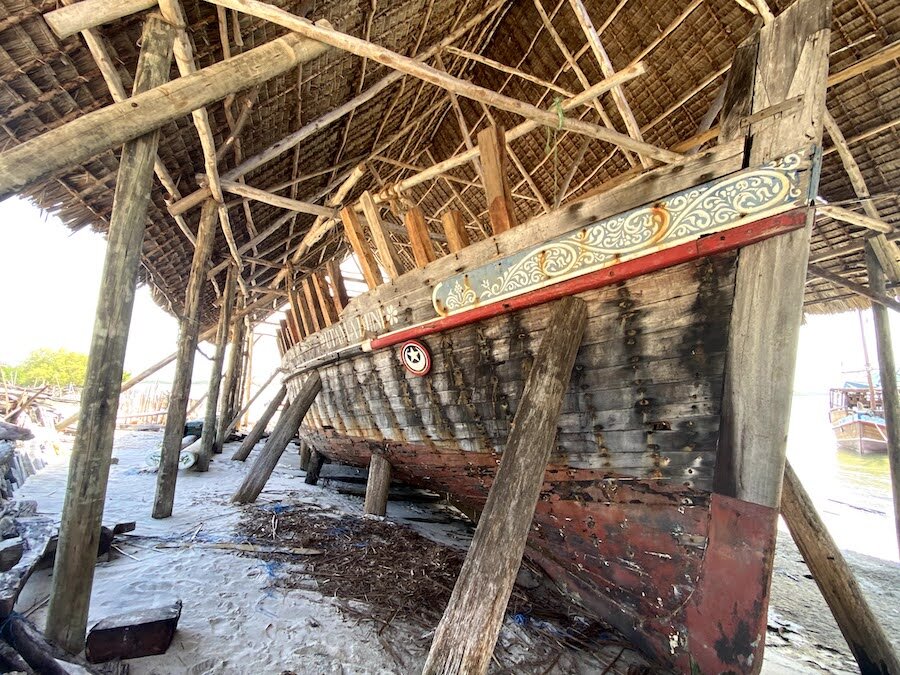The photograph captures an old, weathered wooden boat undergoing restoration, sheltered beneath a rustic thatched canopy supported by wooden poles. Positioned on sandy ground, suggesting close proximity to the ocean, the boat's condition is quite dilapidated, with visible rust around the fasteners of its metal top strap and extensive mold and mildew staining the wood. Additionally, the boat features a distinctive red bottom and an ornate, swirled decorative border around the top, possibly mimicking wave patterns. The boat is supported by various wooden beams on either side, ensuring stability during the restoration process. In the background, there are green trees indicating a warm, sunny environment, along with a glimpse of other boats, hinting at a bustling maritime setting. The scene reflects an area well-versed in boat restoration, with an organized setup for such laborious work.